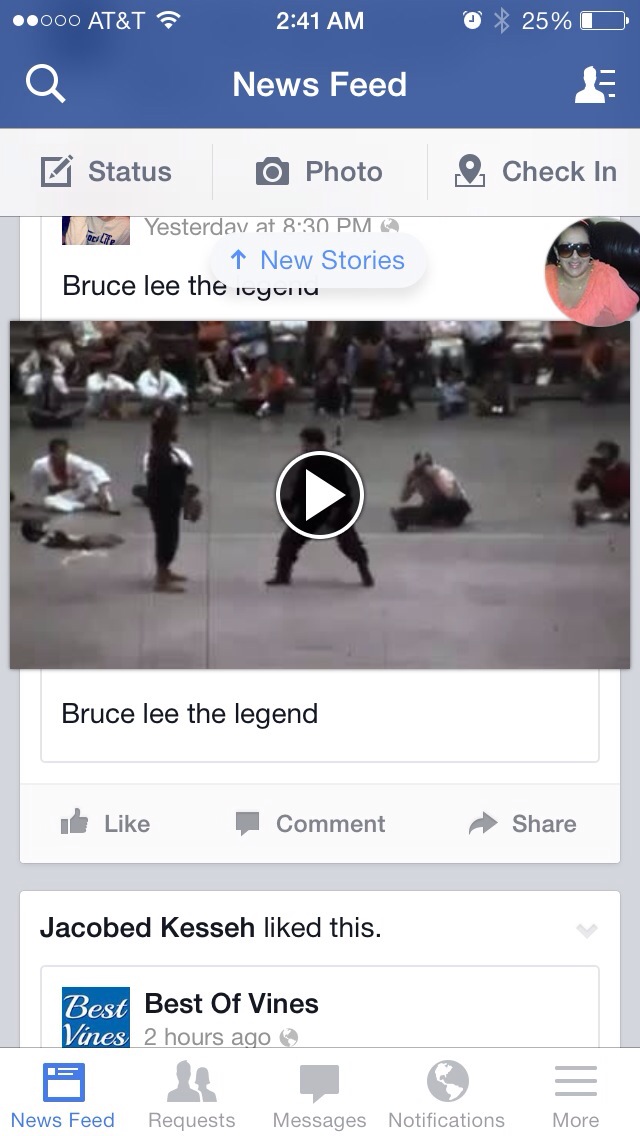This image is a rectangular screenshot of a Facebook newsfeed displayed on a smartphone, captured at 2:41am with the AT&T network showing a 21% battery charge. At the top of the screen are standard phone indicators, including battery strength and signal status. The central focus is a video titled "Bruce Lee: The Legend," which appears to be a martial arts match. Directly below the video, there is a notification stating that "Jacob Kashi likes this," referring to a "Best of Vines" post. 

The top of the feed includes the standard Facebook search bar and the user's profile icon. An up arrow indicating "news stories" suggests that more posts can be viewed by scrolling up. At the bottom of the screen are navigation links for Newsfeed, Requests, Messages, Notifications, and More. The timestamp at the top right next to the AT&T battery indicator shows "Yesterday at 8:30."